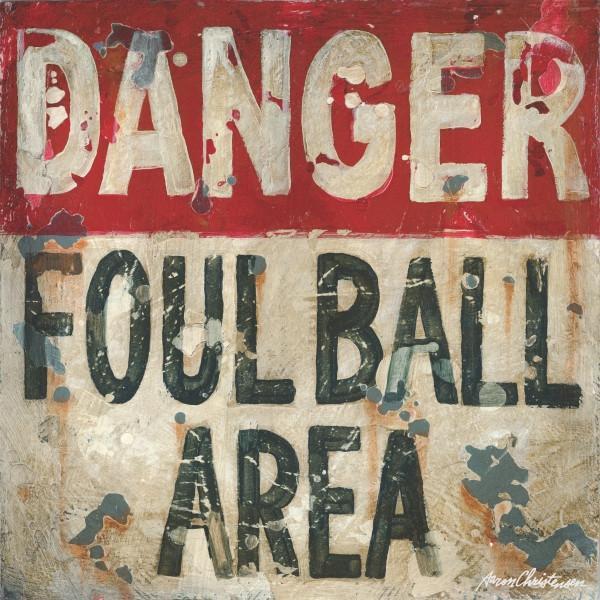The image appears to be an artistically rendered painting of a weathered sign, square in shape, with distinctive features suggesting damage and age. Dominating the upper third portion is a bold red background, upon which the word "DANGER" is prominently displayed in large white block capitals. Below, the bottom two-thirds of the image transitions to a light-colored backdrop with the cautionary text "FOUL BALL AREA" rendered in bold black capital letters. The sign exhibits extensive wear and tear, illustrated through brown stainings, simulating rust, and numerous gray and white splotches mimicking chipped paint. These splotches are sporadic, overlapping the letters and creating a visually distressed effect. The line separating the red top and the light bottom is imperfect, with white paint encroaching into the red area. In the bottom-right corner, a signature in cursive white handwriting can be discerned, likely reading "Aaron Christensen," which suggests the painting might be a modern artistic depiction of a vintage baseball sign.